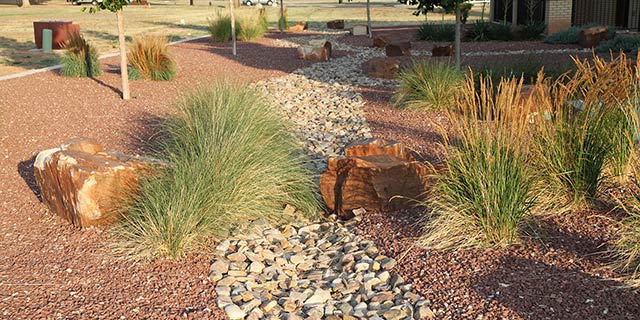This daytime photograph captures an arid garden landscape characterized by a central stone pathway that winds toward the background. The pathway is composed of variously sized and shaped stones in shades of light gray, light brown, tan, and white. Flanking the pathway are patches of small, dark reddish-brown and light brown pebbles interspersed with scrubby desert plants, predominantly green with occasional brown hues. Prominently, two large, medium-brown rocks are situated in the center, with one partially obscured by a bush. Towards the top right, an off-white brick building can be seen in the distance, while the top left features a light green pole and a nearby storage box. The garden also includes spiky green plants growing out of the brown dirt on either side of the pathway. The background hints at a slightly brown field of grass, and additional green, spiky plants continue along the left side, where some trees are planted.